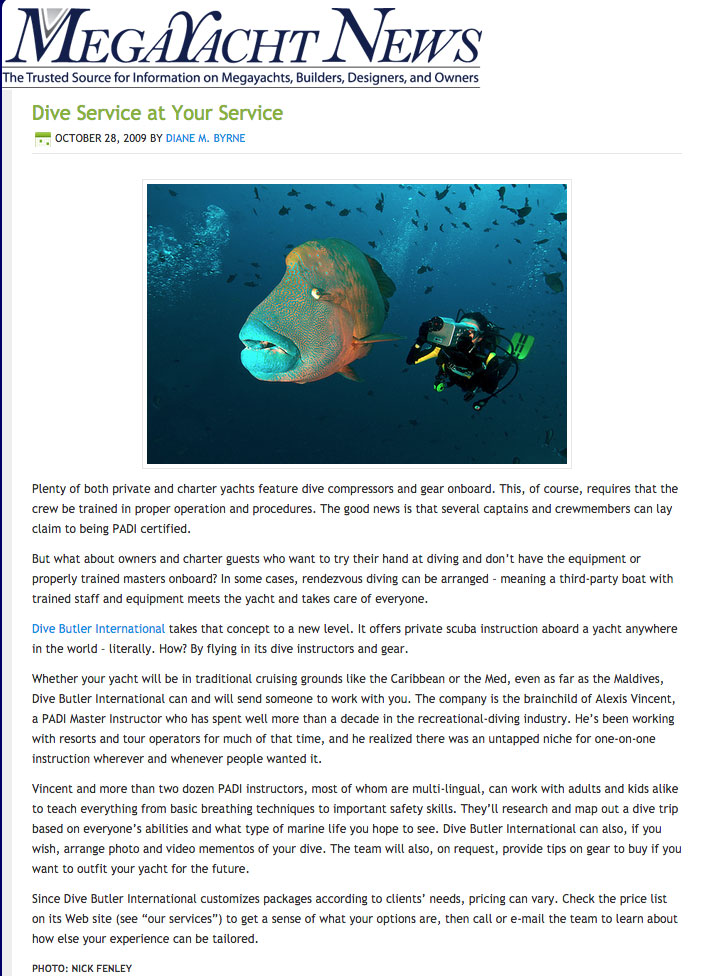**Mega Yacht News: Dive Service at Your Service**

The screenshot showcases a feature on "Mega Yacht News," a website with a white background. In the top-left corner, "Mega Yacht News" is prominently displayed in bold blue letters. Directly beneath this title, a tagline reads, "The trusted source for information on mega yachts, builders, designers, and owners," written in slightly smaller font.

Under this section, a subheading in green lettering states, "Dive Service at Your Service." To the left of the subheading, a green calendar icon appears. Adjacent to the icon, in black text, the date reads, "October 28th, 2009." To the right of the date, in blue letters, the author's name is noted: "Diane M. Byrne."

Centered below, there is a captivating underwater photograph. The vibrant blue water is filled with white bubbles and numerous fish swimming in the background. In the foreground, a large, multicolored fish with light blue lips, a greenish face fading to orange towards its back, and a bulging white eye, takes prominence. Behind the fish, a scuba diver in a black suit with green-striped flippers is visible, possibly holding a camera up to their mask.

Below the image, a detailed article unfolds against a white background with black text. It explains that many private and charter yachts come equipped with dive compressors and gear, which necessitates crew training. Several crew members often hold PADI certification, but it raises the question of what happens when owners or guests wish to dive without proper equipment or a trained dive master on board. The article suggests that rendezvous diving with a third-party boat and trained staff is a solution.

Highlighted in blue letters, "Dive Butler International" is introduced as a service that elevates this concept by offering private scuba instruction aboard yachts anywhere worldwide. They achieve this by flying in instructors and gear. The article elaborates on how this applies to various cruising grounds, from the Caribbean to the Mediterranean and even the Maldives. Dive Butler International is the creation of Alexis Vincent, a seasoned PADI master instructor with over a decade of experience in the diving industry. Vincent identified a niche for personalized, one-on-one diving instruction.

The article continues with more details: Vincent and his team of over two dozen multilingual PADI instructors can teach diving skills to both adults and children, customizing dive trips based on the participants' abilities and desired marine life sightings. They also offer the option to create photo and video mementos and provide gear purchasing advice for clients wishing to outfit their yachts for future dives.

In the final paragraph, the article outlines that Dive Butler International's services are customizable and that pricing varies. For detailed pricing, clients are directed to visit the "See Our Services" page on their website. Readers are then encouraged to contact the team via phone or email to tailor their diving experience further.

At the bottom left of the screenshot, the photo credit reads, "Photo by: Nick Finley."